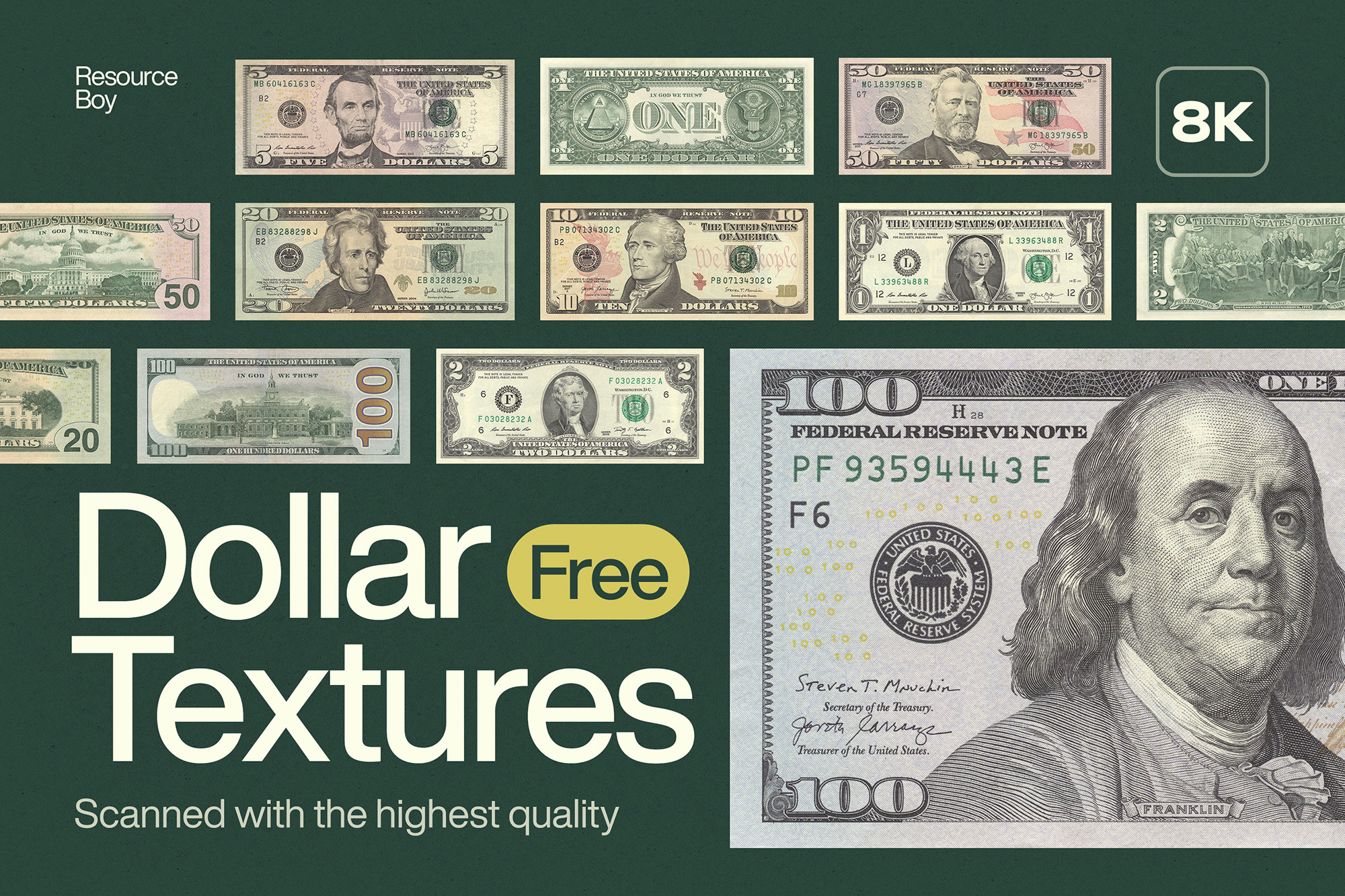This square promotional image, set against a nearly black background, is a high-resolution 8K composite showcasing an array of meticulously scanned, full-color American currency. Top left corner bears the text "Resource Boy" in small white letters, indicating the source. Alongside, you'll find "8K" highlighted prominently. The lower left corner features the phrase "Dollar-free textures scanned with the highest quality." This is a visual array of various U.S. dollar denominations, including front and back views. Specifically, it includes the front of the $1, $2, $5, $10, $20, and $50 bills, and the reverse sides of the $1, $2, $20, $50, and $100 bills. The lower right corner draws attention with a large, partial depiction of Benjamin Franklin from a $100 bill. Together, these elements emphasize the quality and variety of the free dollar textures available for artistic, design, or multimedia projects.